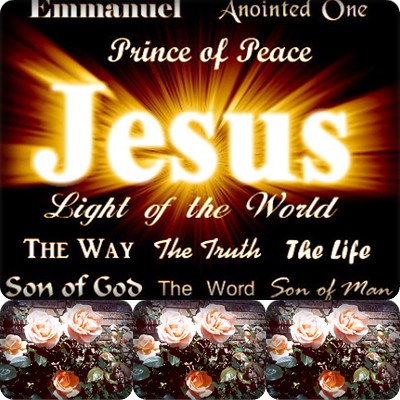The image features a centrally located rectangular sign against a dark black background. The sign prominently displays the name "Jesus" in a bold, bright yellowish-white font, with rays of light appearing to explode outward from it. Above "Jesus," in light cursive script, are the titles "Prince of Peace" and "Emmanuel," alongside "Anointed One" in a lighter, more boxy script. Below "Jesus," in a cursive script, are the phrases "Light of the World," "The Way, The Truth, The Life," and "Son of God, The Word, Son of Man." The text is a mix of cursive and plain fonts, all in white with a golden-white outline, contrasting against the dark background. Beneath this main text area are three identical images. Each image features four light pink roses surrounded by green leaves, set against a stone wall background. These rose images are arranged in a horizontal line, adding a floral element to the otherwise text-dominated composition.